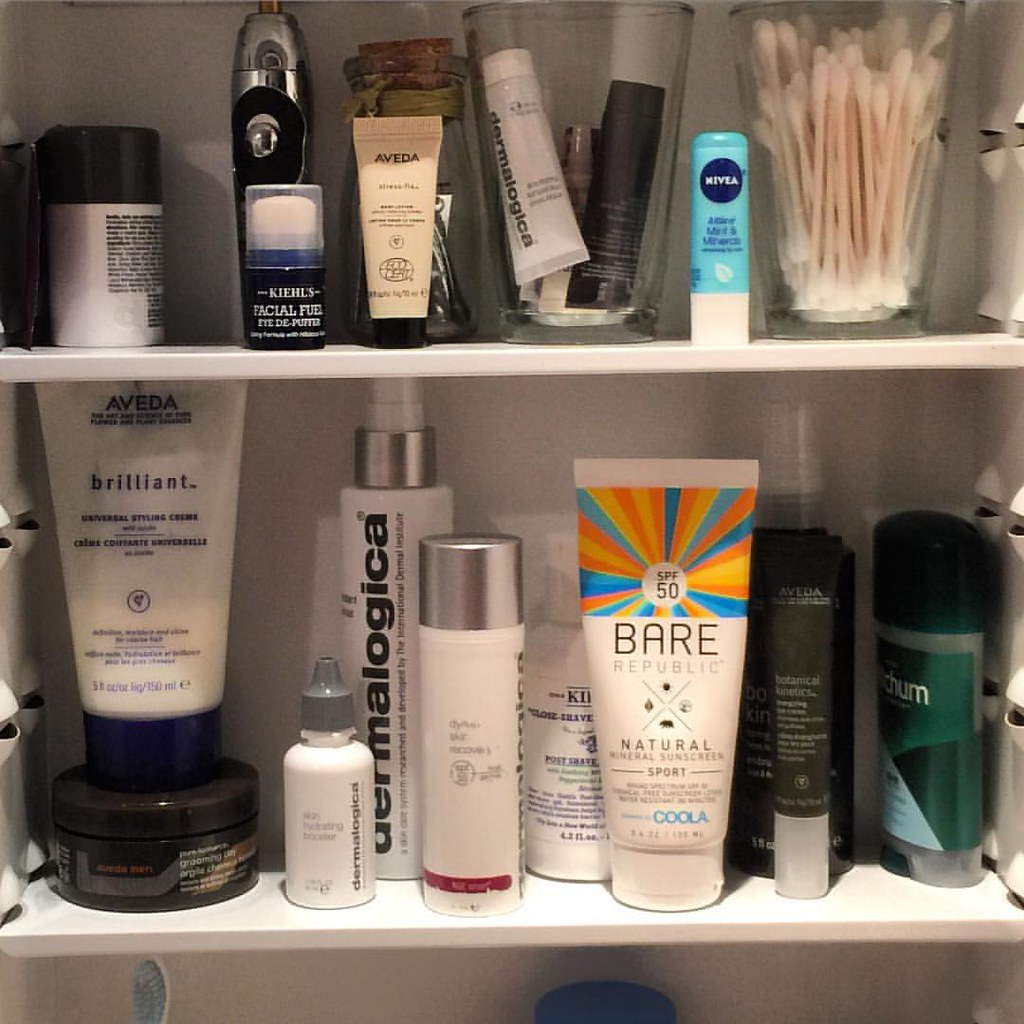This photograph showcases an open medicine cabinet, revealing an organized assortment of personal care items on its shelves.

**Top Shelf:**
1. **Deodorant (Unspecified Brand):** A container with a white bottle and a gray cap, partially turned to reveal fine, illegible print.
2. **Kiehl's Facial Fuel:** A navy blue bottle, presumably an eye cream, with a plastic cap.
3. **Unidentified Metal Device:** Likely battery-operated, featuring a button, though its full structure is obscured.
4. **Aveda Tube:** A container with a flat top, angled design, and a black cap.
5. **Clear Glass Jar:** Topped with a cork stopper, contents inside are not visible.

**Middle Shelf:**
1. **Dermalogica Squeeze Bottles:** Multiple containers from the skincare brand Dermalogica.
2. **Aveda Squeeze Bottle:** Another facial or body care item from Aveda.
3. **Q-tips Container:** A clear container holding a supply of cotton swabs.

**Bottom Shelf:**
A variety of skincare and hygiene products including:
1. **Aveda Lotion:** A bottle of lotion from Aveda.
2. **Bare Republic Sport Sunblock:** A sunscreen product.
3. **Mitchum Deodorant:** A bottle of white deodorant from Mitchum.

Most of the bottles within the cabinet are predominantly white in color, creating a cohesive and organized look to the collection.